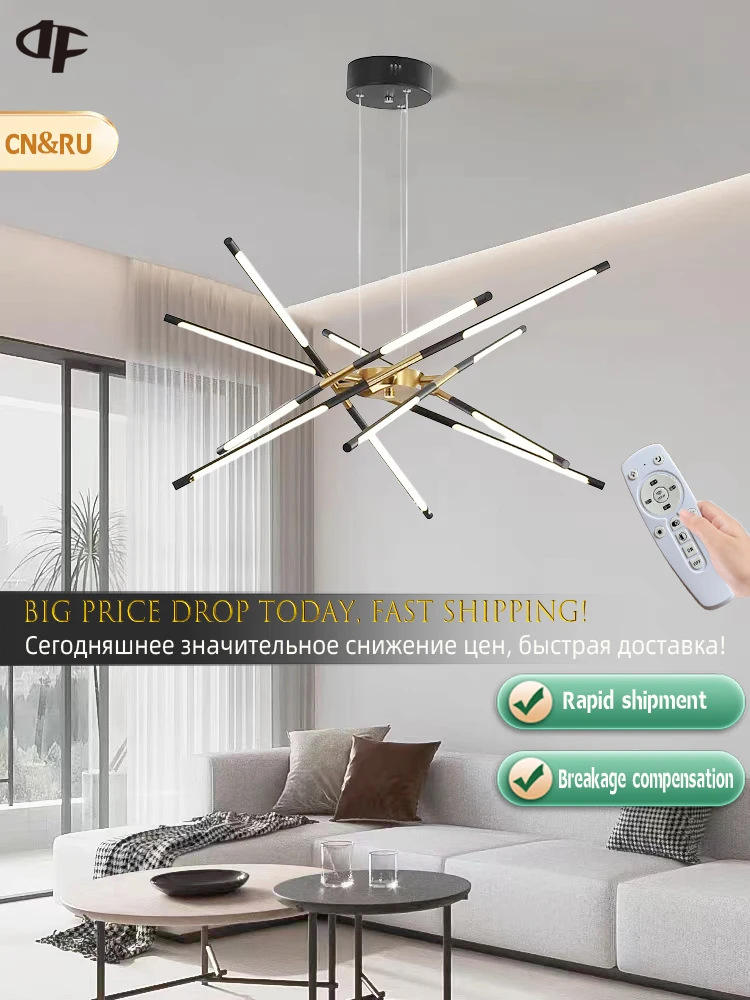The image is a bright and inviting advertisement showcasing a modern, well-decorated living room with a focus on a striking chandelier. The room features a white couch adorned with a brown pillow, a white pillow, a white and black checkered pillow, and a coordinating checkered throw blanket. In front of the couch, there are two coffee tables: a light-colored one with metal legs, topped with a dark bowl, and a smaller, dark table also with metal legs, holding two glasses.

A large sliding glass door on the left-hand side of the room, partially covered by a light white curtain, adds to the room's airy ambiance. The floor appears to be a clean white, harmonizing with the overall bright theme. The centerpiece of the advertisement is an eye-catching chandelier hanging from the ceiling, consisting of long, illuminated bars resembling lightsabers radiating in multiple directions. This chandelier is the focal point, emphasized by a person's hand holding a remote control from the right side of the image.

Promotional text overlays the scene in English and Cyrillic, highlighting "big price drop today, fast shipping." Below this, two green banners with check marks detail "rapid shipment" and "breakage compensation." In the top left corner, a logo featuring the letters "DF" is visible, with a tan oval below displaying "CN & RU" in orange letters, adding a touch of brand identity to the sophisticated setting. The overall atmosphere suggests luxury and convenience, encouraging viewers to take advantage of the attractive offers.